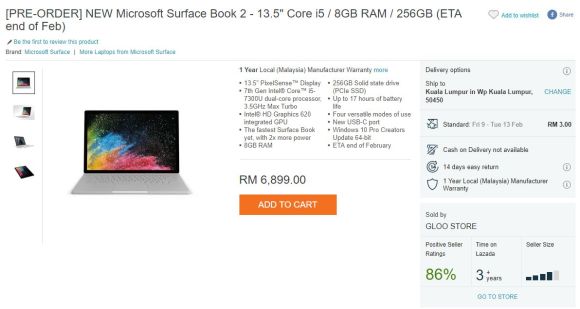**Pre-order** [New]: Microsoft Surface Book 2 - 13.5 inches, Core i5 / 8 GB RAM - 256 GB (ETA End of February)

An image of the Microsoft Surface Book 2 is showcased, displaying its sleek design. The laptop features a black border around the screen, which exhibits an abstract design with splashes of green, blue, orange, and pink colors originating from the corner. The keyboard and base of the laptop are a light silver color. 

Below the pre-order text, there is a pencil icon pointing towards the bottom left, next to the blue text that reads, "Be the first to review this product." 

Underneath, in bold black capital letters, it says "BRAND," followed by "Microsoft Surface" in blue text to the right. 

Dividing each section is a line, under which it mentions "More laptops from Microsoft Surface." 

On the right side, it states "One year local (Malaysia) manufacturer warranty," followed by a blue "More" clickable option for additional information. 

At the bottom of this section, the price is displayed in capital letters as "RM 6,899.00." Immediately below this is a rectangular orange "Add to Cart" button in white uppercase lettering. 

Note: The image quality is low and quite small, making fine details hard to discern.